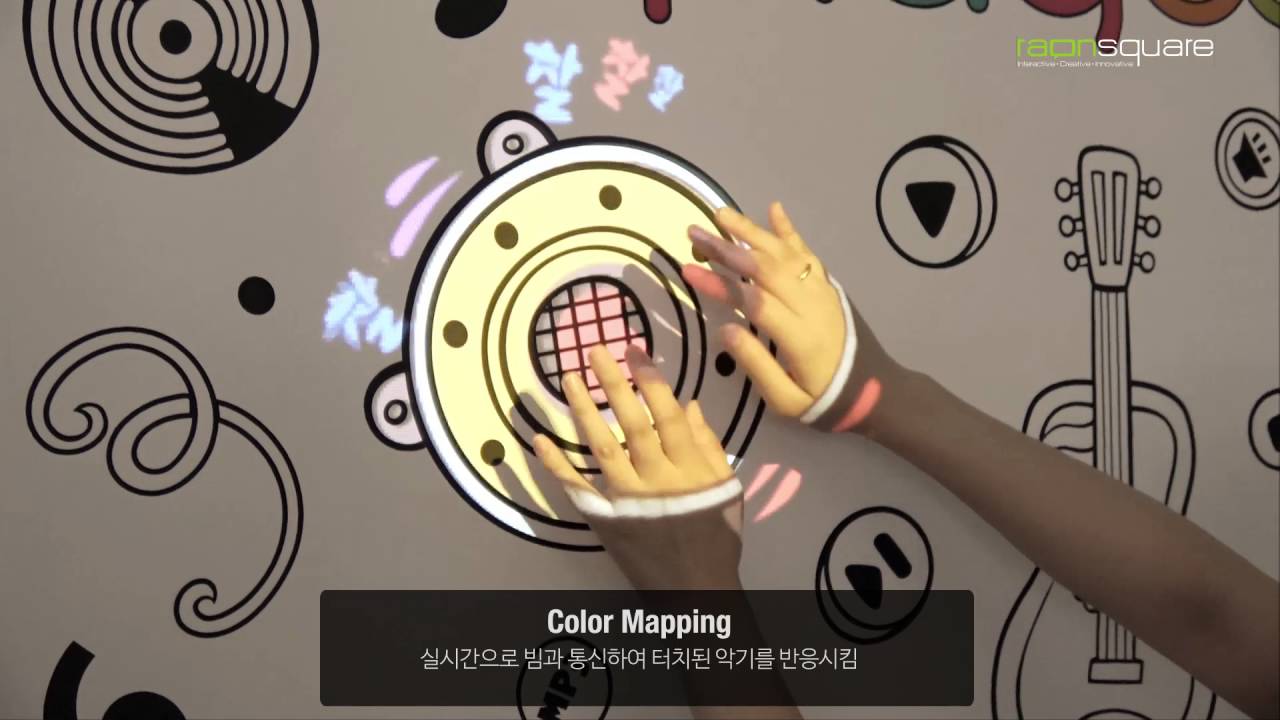The image is a landscape-mode photograph of an artful installation, featuring two light-skinned hands with long brown sleeves and white trims, seemingly tapping a brightly illuminated tambourine. The hands are adorned with a gold ring on the right hand's finger. The background is a taupe-colored wall intricately decorated with various music-themed outlines, including a guitar, circular shapes with grids, vinyl records, squiggly lines, play buttons, speakers, and other sound-related symbols. In the top right-hand corner, the text "RAON SQUARE" is prominently displayed, accompanied by additional text underneath. Below, a large black rectangle with white text reads "color mapping," followed by numerous Asian symbols. The image is vibrant, with bright pink grid lines and a yellow central circle, giving a digital art feel. This could potentially be an advertisement or promotional graphic.